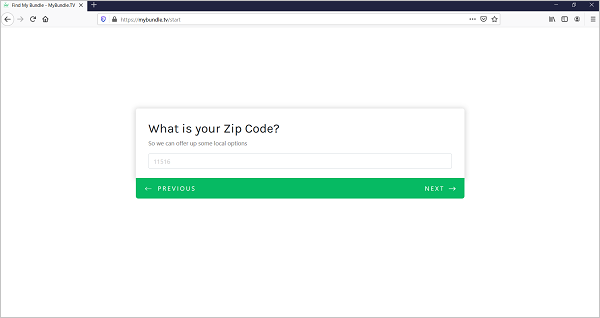The image depicts a web browser interface featuring a predominantly white background. At the center of the page, there is a prominently displayed text box with the question "What is your zip code?" in black text above it. Beneath this question, another line of text is visible but not readable in the image. Directly below this text, there is an input field designated for entering a zip code.

At the bottom of the page, a green navigation bar spans horizontally. On the left side of this bar, there is a "Previous" button accompanied by a left-pointing arrow, while on the right side, there is a "Next" button with a right-pointing arrow.

Additional standard browser elements are visible: an "X" button in the top right corner of both the browser window and the tab, a home button in the top left corner, and other miscellaneous buttons located in the top right area of the browser interface.